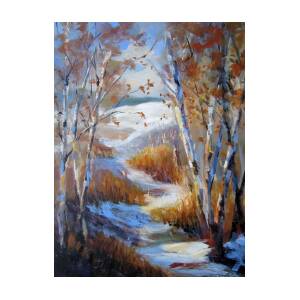The image portrays a detailed oil painting of a snowy autumn landscape, ideal for wall display. In the foreground, a path meanders through patches of snow and brown grass, flanked by tall, slender trees with white bark, reminiscent of birches. These trees display sparse, varying autumn leaves, predominantly red and yellow. The path, shadowed at first, transitions into a sunlit clearing as it recedes into the background. To the left of this path lies a small river or stream that adds a serene element to the scene. The background features a mountain and a light blue sky interspersed with tall, white clouds, enhancing the depth and tranquility of the setting. This low-resolution yet vivid image lacks any visible text or human figures, focusing solely on the natural beauty of the landscape.